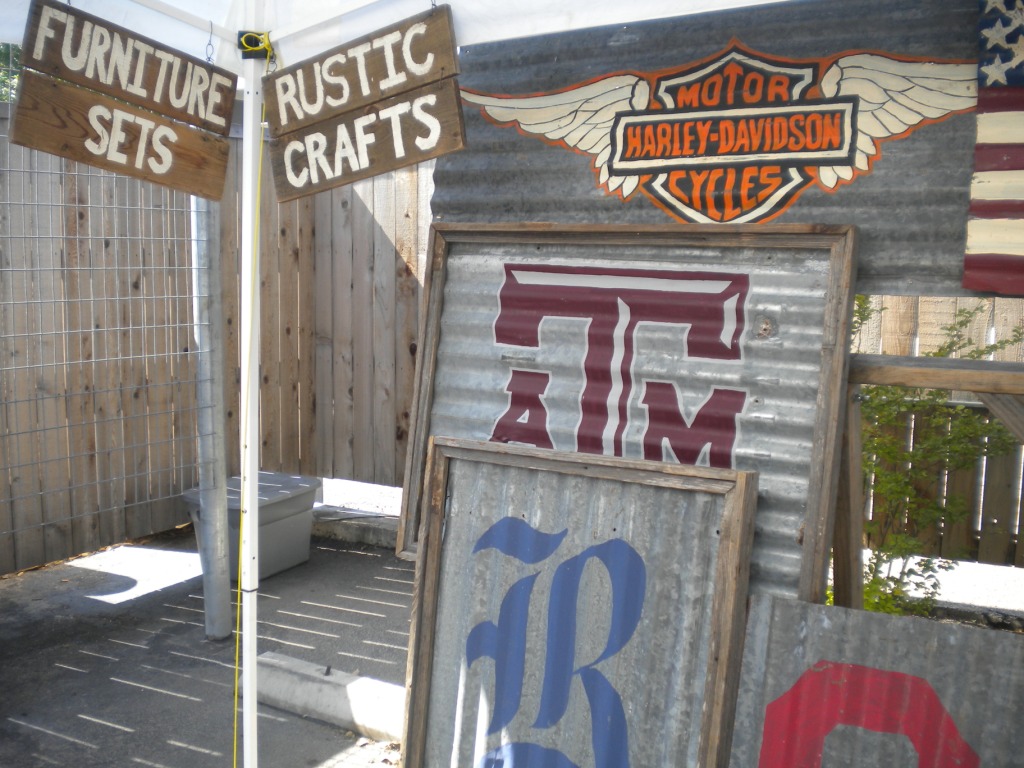In this outdoor photograph, a prominent white pole runs vertically from the top to the bottom of the image. Attached to this pole are several wooden signs: on the left side, there are signs that read "Furniture" and "Sets," while on the right side, signs declare "Rustic" and "Crafts." A wooden privacy fence forms the background, with a gray bucket visible at the bottom near some pavement.

To the right of the pole, a variety of metal signs are leaning against the wooden fence. The uppermost sign features the "Motor Harley-Davidson Cycles" logo, complete with wings extending from the sides. Directly below it is a metal sign displaying a maroon and white "A&M" logo on silver-gray corrugated metal. Further down, another metal sign showcases the letter "B" against a similar background. The collection of signs reveals a mix of rustic wooden and vintage metal designs, adding an eclectic and aged charm to the scene.